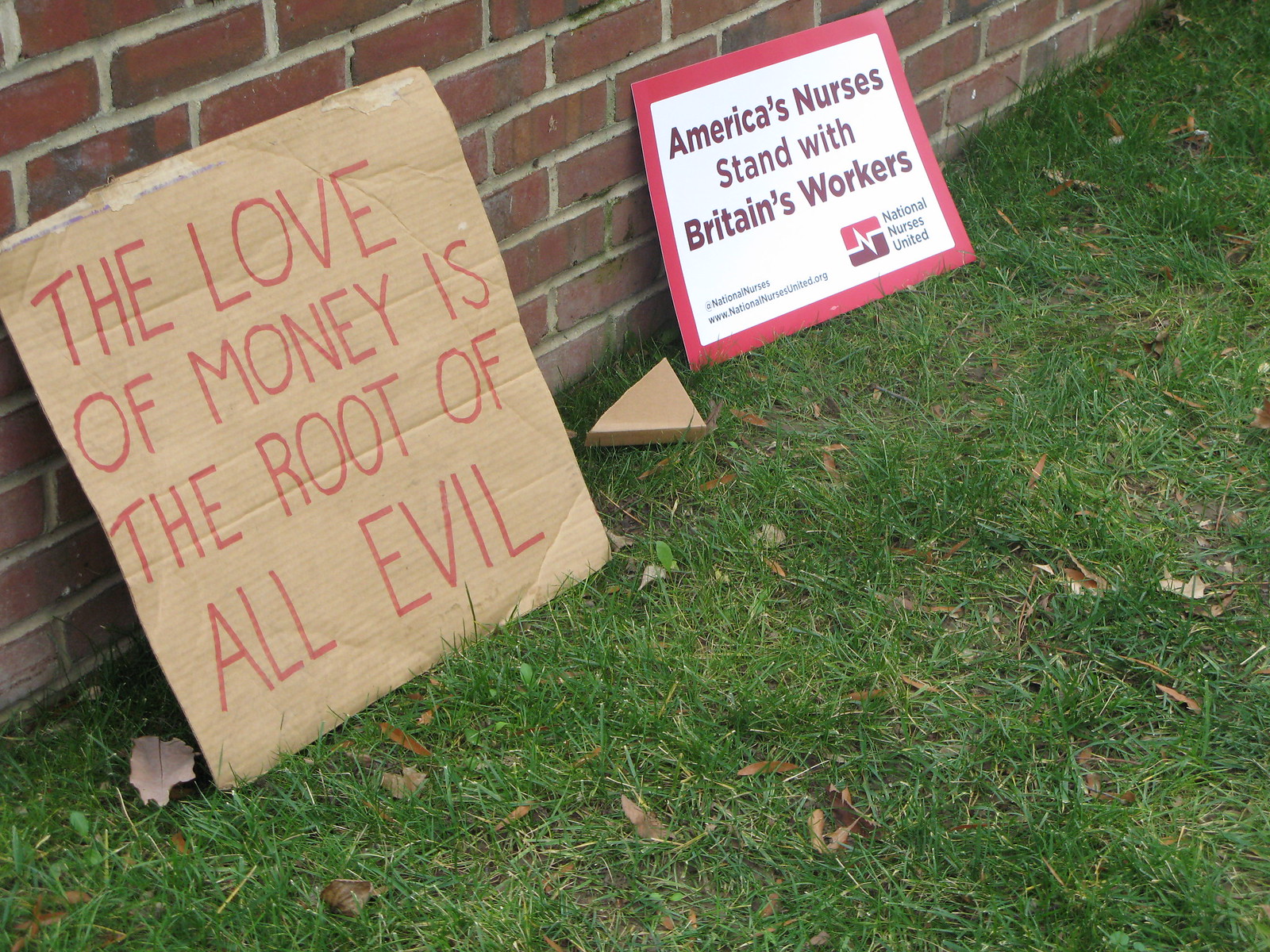In this photograph, we see two signs leaning against an older red brick building. The building provides a backdrop of a diagonal red brick wall that occupies the upper left of the image, while the bottom right half of the image features green grass with a scattering of brown leaves.

The first sign, positioned on the far left, is a square piece of brown cardboard with handwritten text in red, all capital letters. It reads, "THE LOVE OF MONEY IS THE ROOT OF ALL EVIL." This sign adds an organic, handmade quality to the scene.

On the far right side, there is a more formal-looking sign. This sign is white with a bold red border and dark red text in a professional font. It declares, "AMERICA'S NURSES STAND WITH BRITAIN'S WORKERS," and includes a handle, "@NationalNurses," suggesting a social media affiliation. Below this handle, the sign displays a URL, "www.nationalnursesunited.org." Additionally, in the bottom right corner, there's a logo embellished with a maroon and red color scheme and a distinctive white zigzag line representing a heartbeat. The logo is accompanied by the name "National Nurses United."